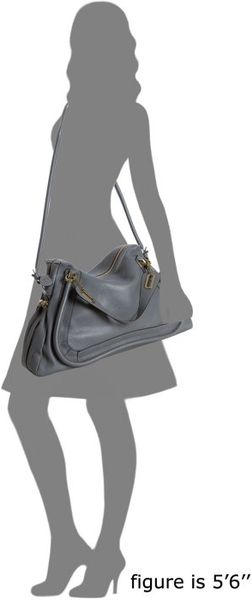The image features a simple, elegant outline of a woman set against an all-white background. The figure, rendered in gray, depicts a woman standing in a poised manner. Her chest faces to the left while her back is oriented to the right. Subtle waves adorn the outline, possibly illustrating hair or a flowing fabric.

The woman's left arm hangs gracefully downwards to her right side, holding a large gray purse. The purse, adorned with small silver or gold notches, rests at her hip and is nearly as wide as her knee-length skirt. A thin strap spans across her right shoulder, complementing the overall minimalist aesthetic.

Her legs, outlined definitively, show her right leg slightly forward, with its heel lifted and overlying the left foot, which is firmly planted flat on the ground. She wears high heels, adding to her stylish appearance. To the right of the figure, bold black lettering indicates her height as "5'6"." The professional, monochromatic design gives the image a neat and sophisticated look.